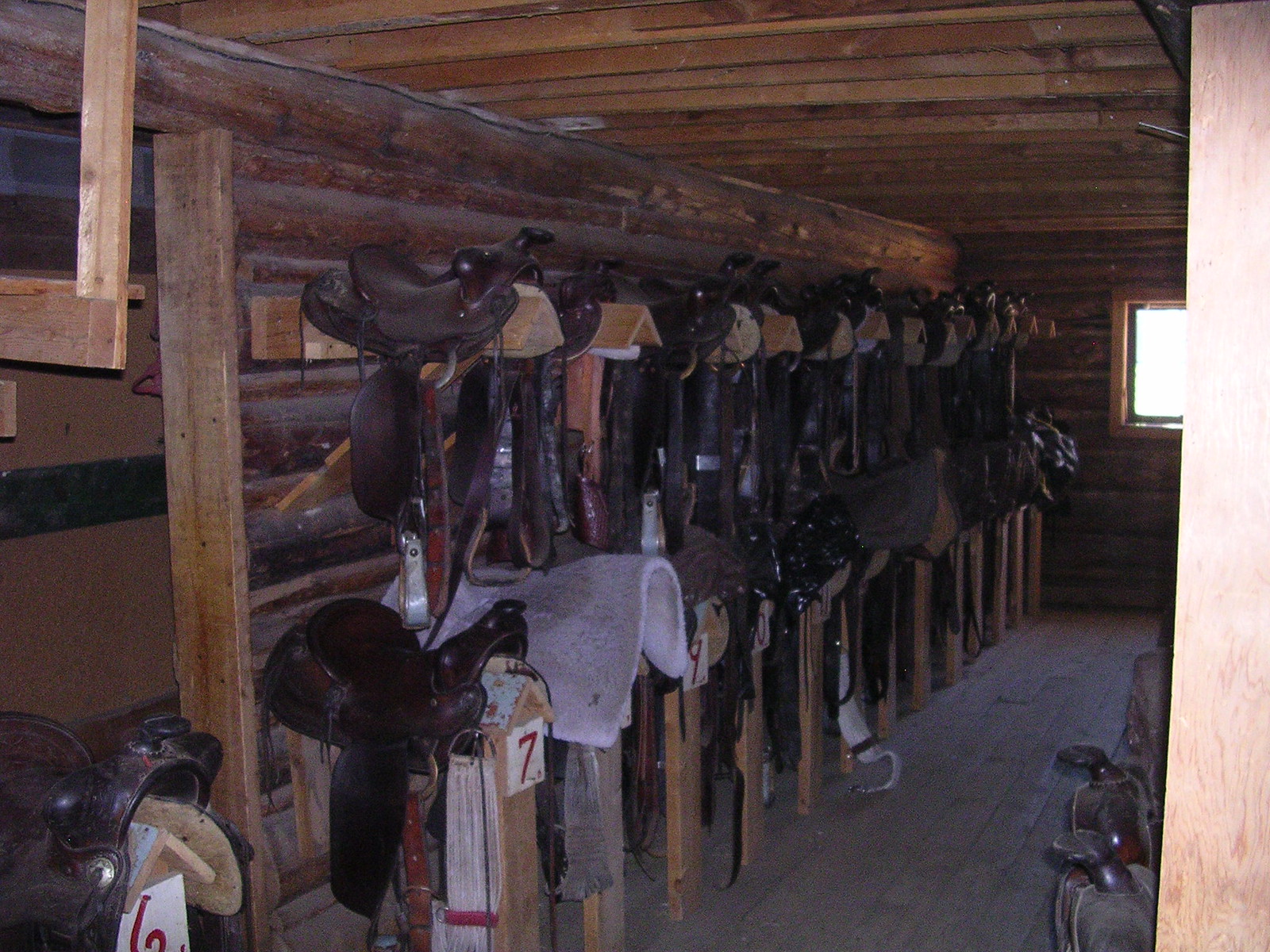The image depicts the interior of a rustic wooden structure, which appears to be an attic, barn, or equestrian storage hut. The floor, walls, and ceiling are composed of wooden beams and planks. A small window on the right side of the frame allows some light into the otherwise dimly lit space. The focal point of the image is a series of horse saddles arranged in two rows on wooden poles. Each pole in the bottom row features saddles marked with numbers on white cards in red ink, ranging from 6 to 11. The top row also displays leather saddles, though they lack the numbered labels. The overall atmosphere is somewhat dark, possibly due to the exposure contrast with the sunlight filtering in through the window.